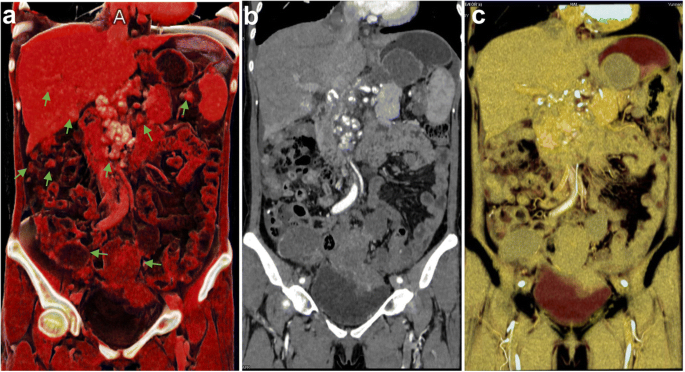This wide rectangular image is divided into three equal sections labeled A, B, and C, showcasing what appear to be repeated paintings of an oddly shaped creature adorned with a headscarf or mask and intricate jewelry attached to varied fabrics. Each section, highlighting different color schemes and details, resembles an x-ray view of a torso from above the knees to the base of the skull. 

- Section A, on the left, is predominantly red and black with neon white elements at the bottom resembling bones; it also features small green arrows within the figure.
- Section B in the center, displays the figure in shades of gray with silver accents, offering a monochromatic view.
- Section C, on the right, is primarily yellow with noticeable red and black splotches, particularly near the legs and the right shoulder.

The image presents an intriguing portrayal as if examining the same subject under different conditions or highlighting diverse aspects, unified solely by the bold letters A, B, and C in the top left corner of each section.